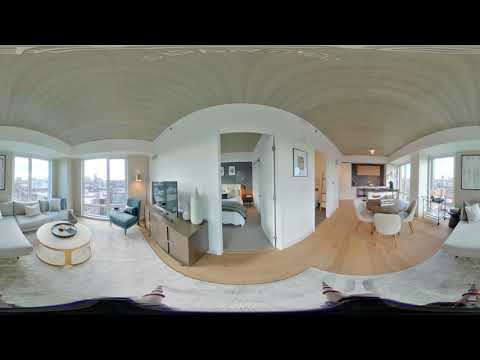The image depicts a panoramic view of a modern city apartment, capturing multiple areas within an open layout. Starting from the left, a living room features a light gray couch with several pillows under a framed picture or painting, adjacent to a round coffee table. Large windows along this wall offer expansive views of the city, enveloping a sitting chair positioned beside one of the windows. The ceiling has a plaster finish, adding to the room's sophisticated appearance.

Moving to the center, there's a TV mounted on a wooden hutch with compartments below, some vases, and two large cabinets. Beside this setup is a door leading into a curved bedroom, visible with its bed, gray carpet, and blue walls.

To the right of the bedroom, the open space flows into a dining area, delineated by a light beige floor, contrasting with the adjacent white carpet. The dining area features a table surrounded by three or four white chairs. The room extends to the right with more windows that continue to showcase the urban landscape outside. The cohesive layout, enhanced by the panoramic perspective, reveals a spacious and well-lit apartment, possibly staged for sale or display.